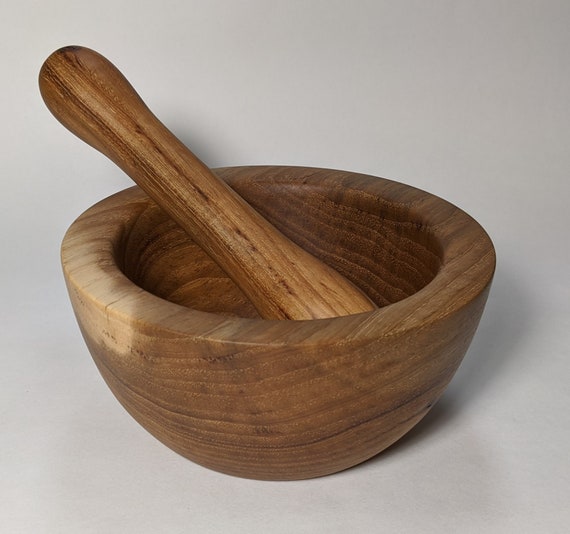This photograph features a wooden mortar and pestle set used for grinding herbs, spices, salts, and other cooking ingredients. Both pieces are crafted from what appears to be oak or a darker spruce wood, finished with a medium brown stain that highlights their natural grain. The pestle, roughly 8 inches long, has a drumstick shape, while the mortar, with a diameter of about 6 inches, is bowl-shaped. The set shows some signs of use and aging, notably a faded spot on the top left lip of the bowl where the finish has worn off. The background is a gray-to-white gradient with warm undertones, enhancing the earthy richness of the wooden pieces. The photograph solely features the mortar and pestle, with no additional text or objects.